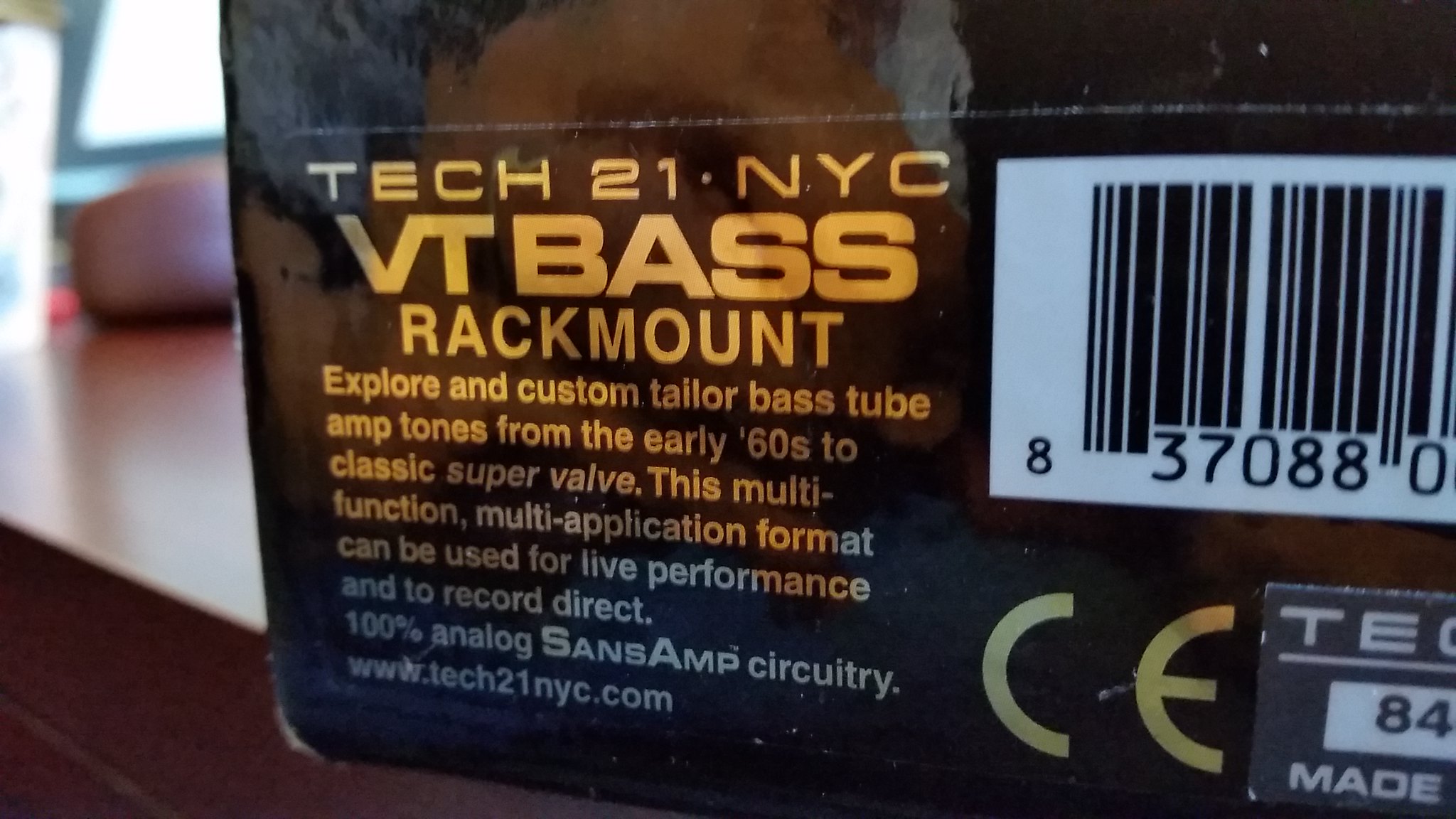This image features a prominently displayed black box with a gray or silver text that reads "Tech 21 NYC VT Bass Rack Mount." The box occupies the central portion of the image, attracting most of the viewer's attention. To the left, a table is partially visible, adding context to the setting. The detailed text on the box indicates that it is designed for exploring custom-tailored bass tube amp tones from the early '60s to classic Super Valve sounds. This multi-functional, multi-application device can be used for both live performances and direct recording, boasting 100% analog SansAmp circuitry. The bottom right corner of the box has additional logos or stickers, while the right side features a partially visible barcode and logos that appear to include a "C" and an "E." For more information, the box provides a web address: www.tech21nyc.com.